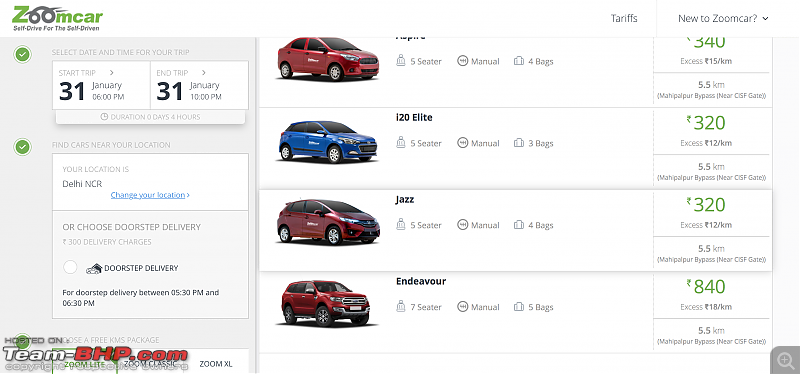The image displays a detailed screenshot of a business page for selling cars titled "Zoom Car." The logo, positioned in the upper left, features a capital 'Z' in green, with the 'OO' stylized to resemble a car zooming away in black or gray. The remaining lowercase letters 'mcar' are in green, and the logo is accompanied by the tagline "Self-drive for the self-driven."

Underneath the logo, there are two sections with checkboxes ticked in white within green circles. The first checkbox is for selecting the date and time for the trip. It states:
- Start Trip: 31st of January at 6 p.m.
- End Trip: 31st of January at 10 p.m.
- Duration: 0 Days, 4 Hours.

Following this information is a section titled "Find Cars Near Your Location." It indicates:
- Your Location: Delhi NCR
- Optional hyperlink: Change Your Location (in blue).

Additionally, there is an option for doorstep delivery, stating:
- Doorstep Delivery: ₹300 delivery charges
- Delivery Time: Between 5.30 p.m. and 6.30 p.m.
- Icon: Small car in front of a house, circle not filled.

At the bottom, a note mentions that the page is "Hosted on TeamBHP.com," with 'Team' in white and 'BHP.com' in red, partially obscuring background information. The background also contains the text "Zoom XL."

On the right side, four cars are displayed, each facing right with their fronts and rears directed. The details are as follows:
1. **Top Car (Red)**
   - Type: Four-door sedan or compact car
   - Capacity: 5-seater
   - Transmission: Manual
   - Luggage: 4 bags
   - Price: ₹340
   - Excess: 15 kilometers
   - Location: 5.5 km from Mahipalpur Bypass near CSF Gate.

2. **Second Car (Blue)**
   - Model: I-20 Elite
   - Capacity: 5-seater
   - Transmission: Manual
   - Luggage: 3 bags
   - Price: ₹320
   - Excess: 12 kilometers
   - Location: 5.5 km from Mahipalpur Bypass near CSF Gate.

3. **Third Car (Red)**
   - Model: Jazz
   - Capacity: 5-seater
   - Transmission: Manual
   - Luggage: 4 bags
   - Price: ₹320
   - Excess: 12 kilometers
   - Location: 5.5 km from Mahipalpur Bypass near CSF Gate.

4. **Bottom Car (Red and Silver SUV)**
   - Model: Endeavour
   - Capacity: 7-seater
   - Transmission: Manual
   - Luggage: 5 bags
   - Price: ₹840
   - Excess: 18 kilometers
   - Location: 18 km from the user's current position.

There is no other visible text, and the page provides a clear, structured overview of car rental options and associated details.